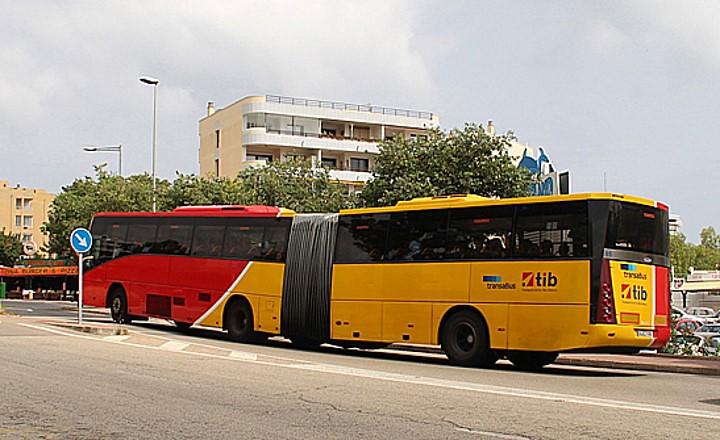The photograph captures a scene of a large, articulated bus on a city street. The bus comprises two sections connected by a black accordion-style flexible joint. The front section is predominantly red with yellow accents, while the rear section is primarily yellow with a red stripe and features the logo and name "Transabus" and "T-I-B." The windows of the bus are darkly tinted, obscuring the view inside, though silhouettes of chairs and possibly passengers are slightly visible. The bus has a total of six wheels, with two visible at the front and one at the rear. The street is marked with white and blue lines indicating lanes, and the pavement features a blue arrow pointing to the right.

Behind the bus, a mid-rise yellow building with white-striped balconies stands amidst a landscape of trees with visible green leaves. The sky above is a muted blue-gray, dotted with fluffy clouds, suggesting an overcast yet clear day. The surroundings hint at a smaller town or city setting, with additional smaller buildings and apartments in the background. Also visible are parked cars—a red car and a white car—adding context to the urban environment. The bus dominates the scene as it travels along the gravel-lined road, framed by street lights and other city infrastructure.